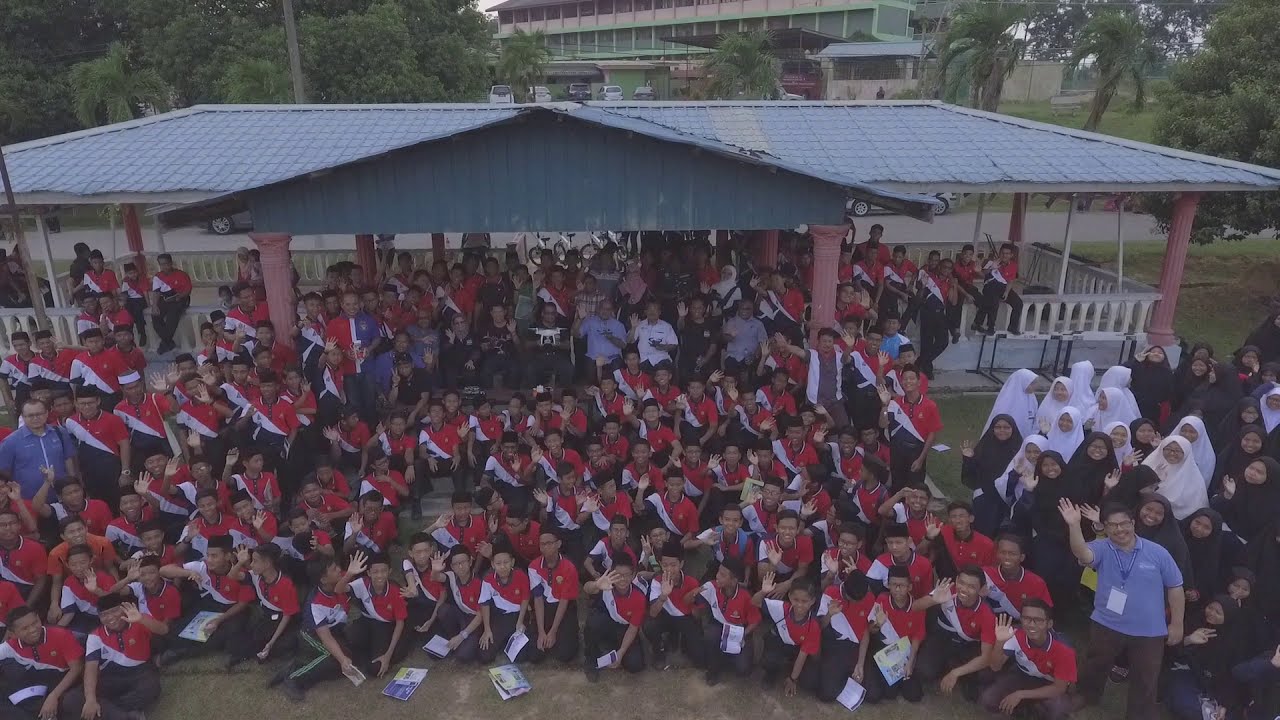In this colorful, high-angle drone photograph, a large group of almost 100 people is assembled in a courtyard and steps of a structure with a blue roof, supported by red columns, and a white banister around the edges. The group predominantly consists of children wearing matching uniforms featuring red diagonal shoulder sections, white diagonal stripes across their chests, dark pants, and holding white papers with a dark rectangle. The children are seated in the center, with adults positioned on the right, left, and towards the back. Most of the children and adults are waving and smiling towards the camera. In the lower right corner, a group of women in white and black hijab veils with matching robes and a man in a blue t-shirt with a hang tag ID, possibly a coach or instructor, can be seen smiling and waving at the camera. Palm trees frame the scene on the left and right sides. The style of the photograph is representational realism.